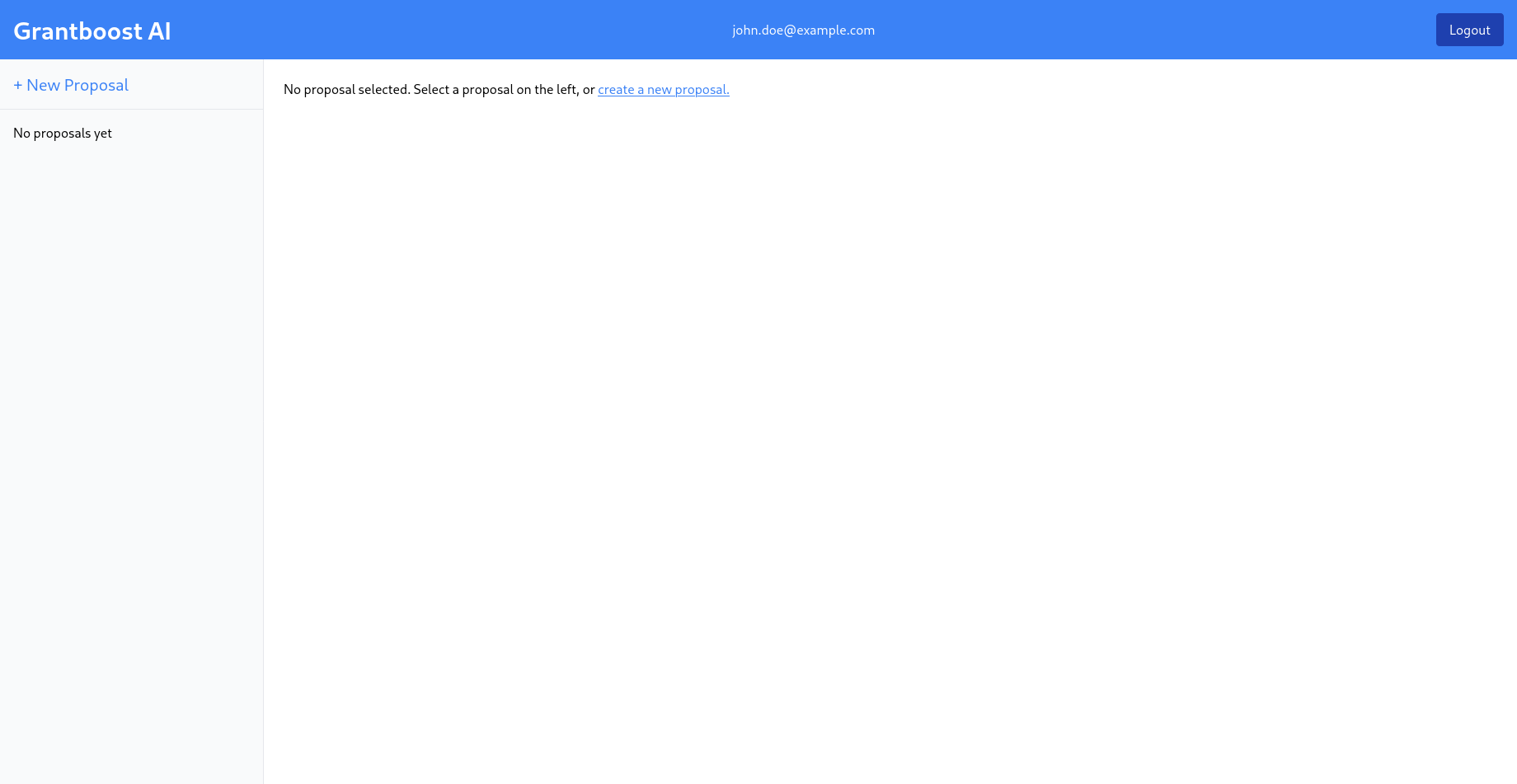The image appears to be a computer screenshot displaying an interface of a software or web application named "Grant Boost AI". At the top, there's a blue banner with the title "Grant Boost AI" on the left side in white text, and in the center, the user’s email address "JohnDoc at example.com" is visible. On the far right corner of the banner is a dark blue button labeled "Log Out" in white text.

The left side of the screen features a light gray sidebar. At the top of this sidebar, the text "New Proposal" is displayed in blue, and directly beneath it, the words "No Proposals Yet" are written in black.

The main part of the screen, occupying the right side, is predominantly white. Here, in black text, it reads "No Proposal Selected". Below this, there is an instruction in black text: "Select a proposal on the left or create a new proposal." The phrase "Create a New Proposal" is highlighted in blue and underlined, indicating that it is a clickable link.

The layout is very clean with no images or pictures; it mainly consists of text elements. The background remains primarily white, with the majority of the text in black, and selected actionable items in blue.